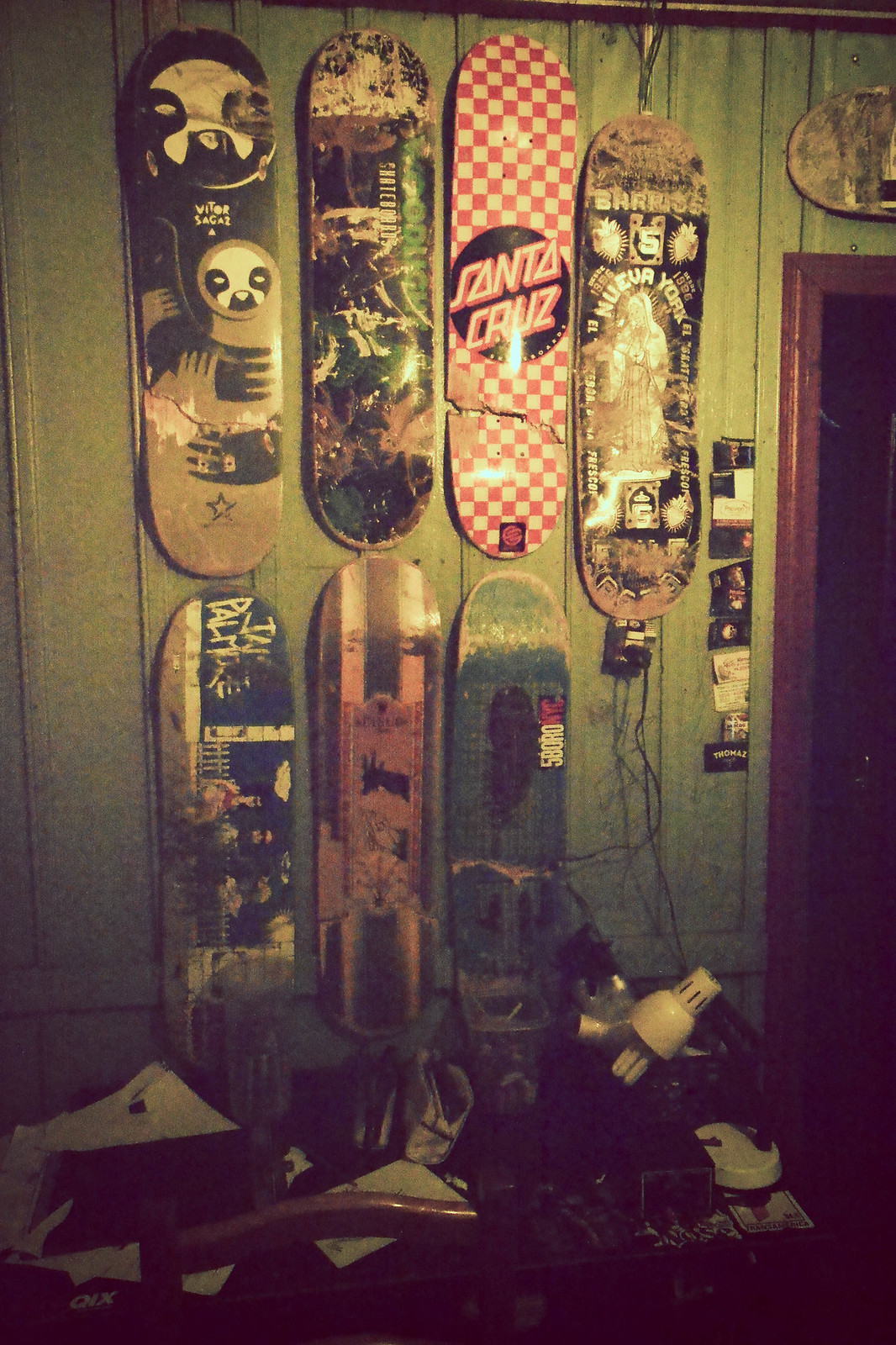This photograph showcases an olive green paneled wall adorned with seven skateboard decks arranged in two rows. Each deck boasts intricate patterns or graphics, though the muted, grainy quality of the image with its greenish cast adds a vintage feel. In the upper row, starting from the left, the first skateboard features text that reads "Vitor Sog," accompanied by cartoon characters—a black figure embracing a tan one. Next is a distressed board in browns, blacks, whites, and greens. The third deck is a striking red checkerboard pattern with a black circle and the iconic "Santa Cruz" logo in futuristic red and white lettering, visibly cracked from wear. The fourth top board appears to feature metallic tones, with "Nueva York" text and an angelic figure, possibly the Statue of Liberty, though poorly lit. In the lower row, the decks are even more worn but display a variety of distressed, colorful designs. Notably, one bears white text, though it is illegible. To the right of the wall is a partially visible brown door frame. The floor beneath the wall is cluttered with indistinct objects, including what looks like a white lamp head, contributing to the dim, chaotic ambiance of the scene.